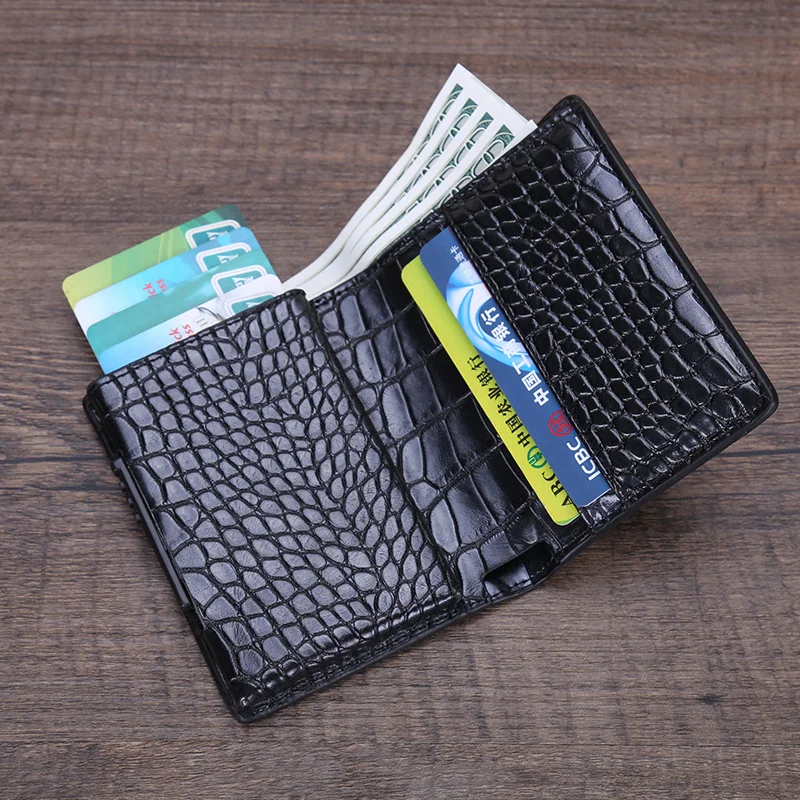This detailed photograph features a black wallet, designed to resemble alligator or snake skin, resting on a rustic wooden table with prominent wood grain. The wallet is open, revealing its contents. On the right side, two plastic cards are visible, including a fluorescent green card labeled "ABC" and a blue card labeled "ICBC" with Chinese writing. At the top of the wallet, four $100 bills are slightly poking out, just enough to identify their denomination. To the left of the cash, there are four cards fanned out, displaying light blue, teal, light blue, and fluorescent green colors. The table, in good but purposefully rustic condition, serves as the backdrop for this arrangement of everyday essentials, showcasing the wallet's shiny texture that might suggest either genuine leather or a vinyl imitation.